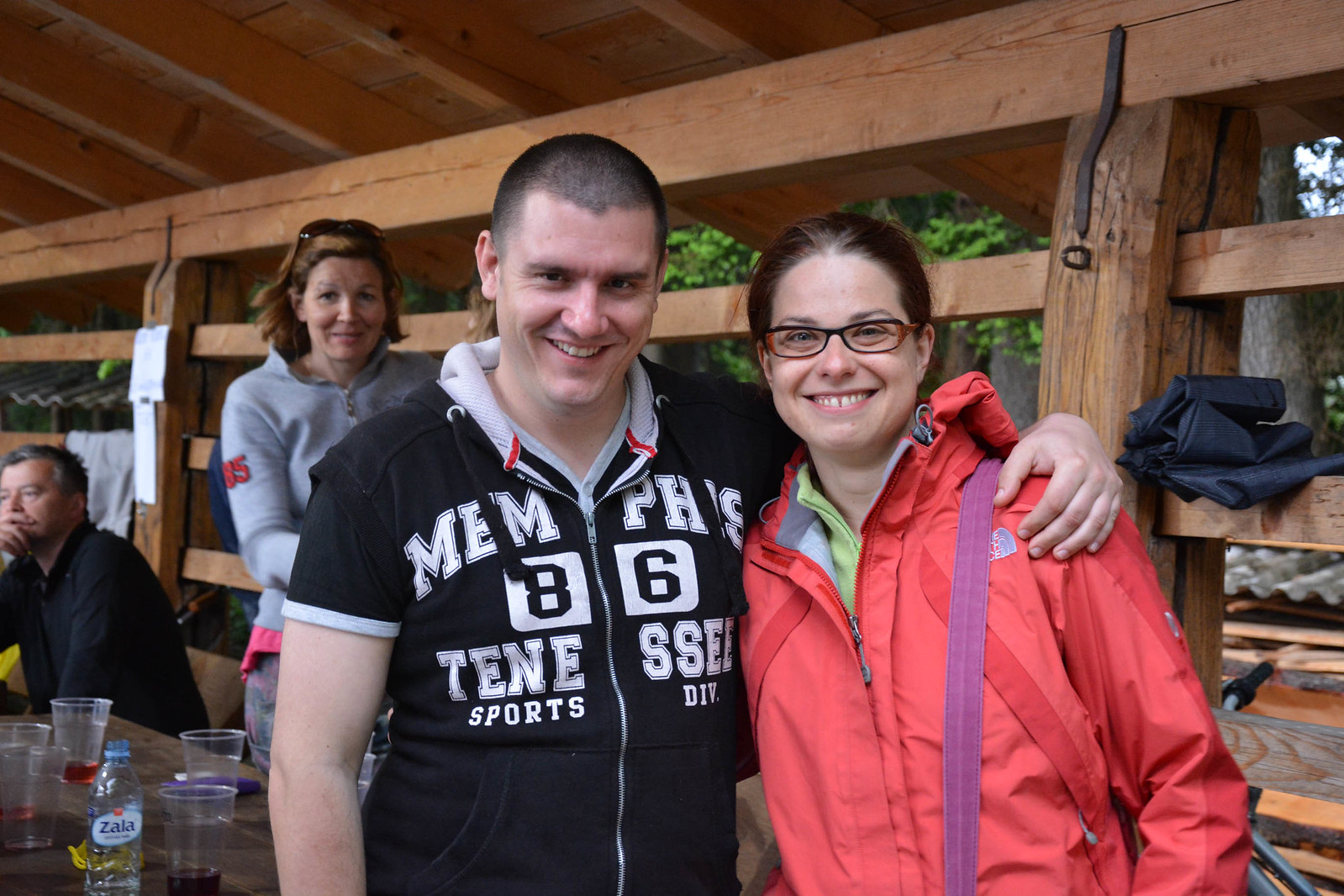The image captures a happy moment featuring a man and a woman smiling directly at the camera. The man, of decent build with short black hair and a big smile, is dressed in a black short-sleeve hoodie emblazoned with "Memphis 86" in white lettering. He has his arm around the woman beside him, who is sporting a reddish-pinkish North Face jacket, with long brown hair and glasses. She also has a purse draped over her arm. In the background, there are other people: a man staring off into the distance and an older woman, with a table nearby holding mostly half-drunk drinks. They appear to be inside a large wooden structure, possibly a pavilion, characterized by wooden beams and shelves that frame the setting.